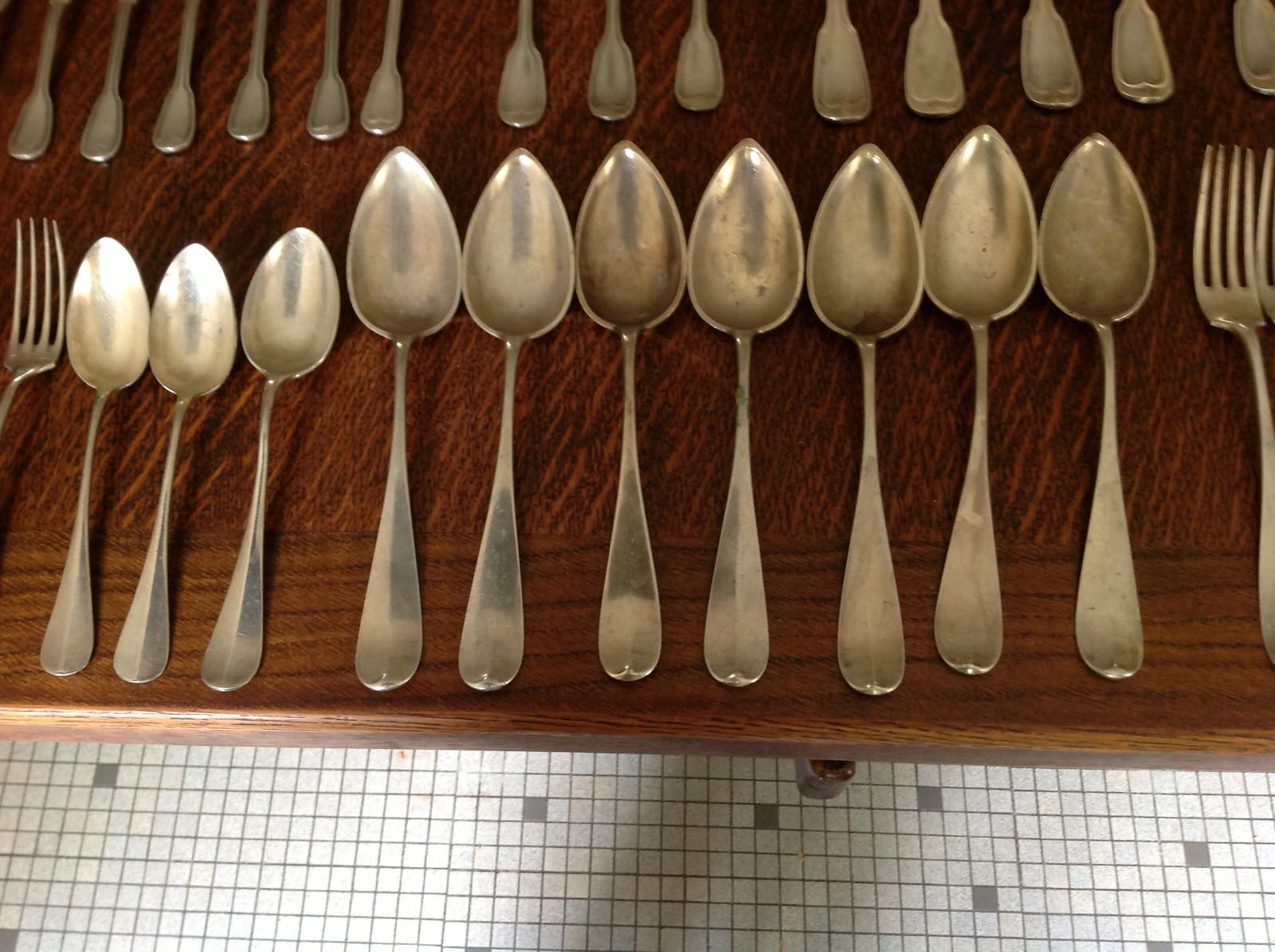The image is a color photograph capturing a collection of silverware displayed on a medium brown, richly toned wooden surface. The wood rests on a white and gray checkered tile floor. On the wooden surface, the arrangement starts on the left with a single four-tined fork, followed by three plain silver teaspoons. Next to the teaspoons are seven plain silver tablespoons. On the far right, another four-tined fork is positioned. Above this neat array, the bases and stems of additional pieces of silverware are visible, although it's unclear whether they are forks, knives, or spoons. The silverware does appear somewhat tarnished, suggesting it might need polishing. This detailed display might be part of a personal collection, perhaps being shared, sold, or recently acquired.